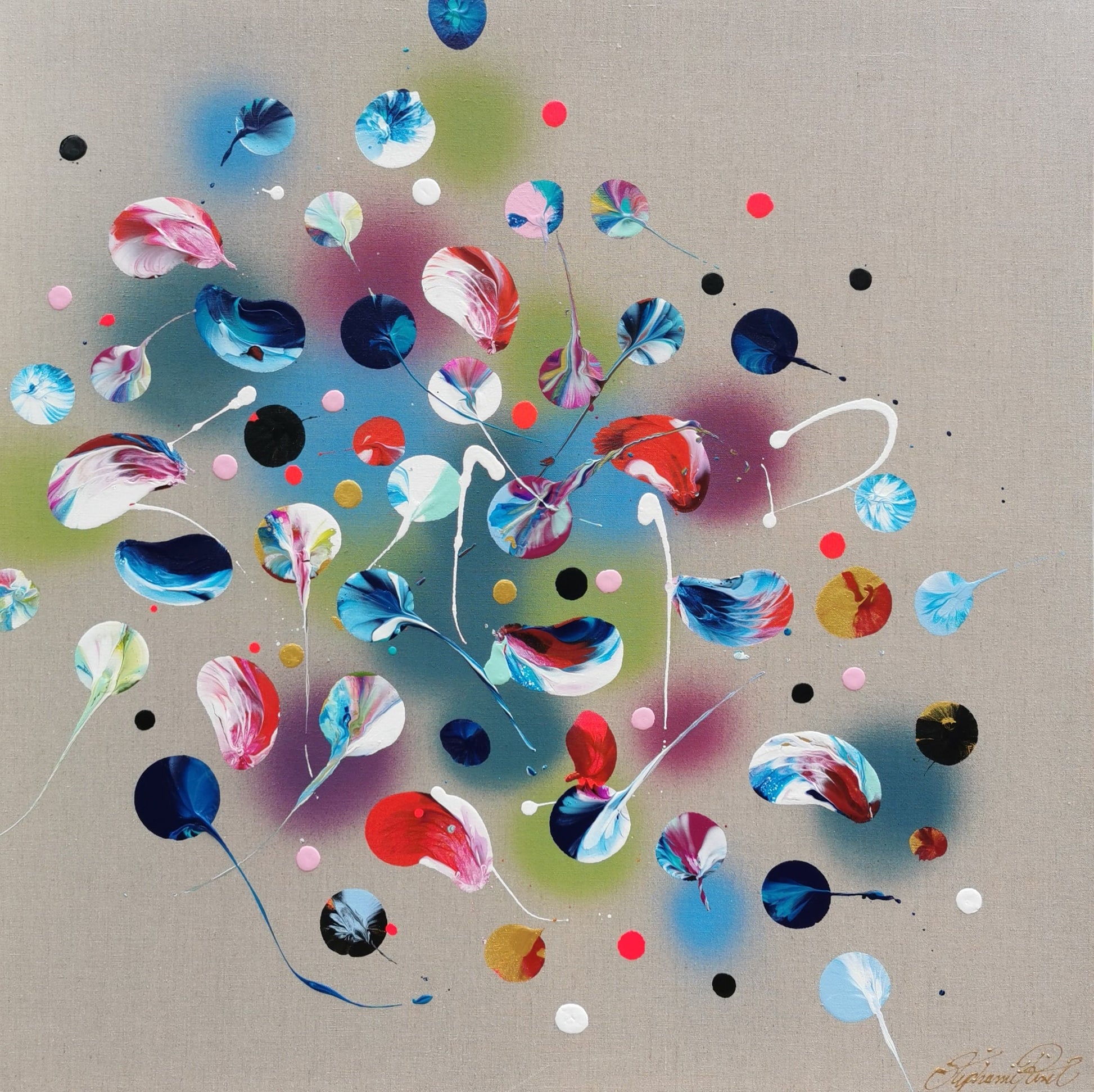This artwork features an abstract composition characterized by an array of vibrant, feathery blossoms in diverse colors, including electric blue, red, white, mint green, and purple. These blossoms, resembling feather shapes, appear to be cascading across the piece, creating a dynamic movement. The background is a subtly textured gray canvas, lending a sense of depth and contrast to the vivid colors in the foreground. This layered effect is enhanced by the soft blur of the background, allowing the more defined and colorful blossoms to stand out prominently. Additionally, the art piece includes what appears to be a signature or text—possibly "Stefanik's pole"—adding an enigmatic touch. The overall setting resembles a canvas or similar material, making it a striking example of interpretive, abstract painting.